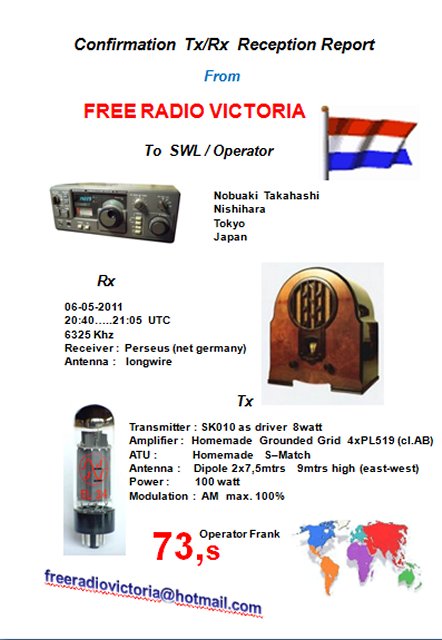The image is a screenshot of a reception report from Free Radio Victoria, addressed to 2SWL operator Nabuaki Takahashi in Tokyo. It showcases a confirmation of TX (transmitter) and RX (receiver) reception, filled with technical details. At the top of the document, a colorful header features Free Radio Victoria's logo, and a flag in red, white, and blue, though its specific reference is unclear.

The middle section displays various radio devices: on the left, an image resembling a boombox, representing the receiver, and an even older radio device on the right, possibly signifying historical equipment. Accompanying these images are technical specifications, such as the receiver type (Perseus in Germany), antenna type (long wire), transmitter details, amplifier specifications, and modulation techniques.

At the bottom of the image, there is a flattened, colorful map of the world, emphasizing the global reach of Free Radio Victoria, along with their contact information at Hotmail.com. Despite the modern and vibrant appearance, the image quality is somewhat low, suggesting it might be a scan or screenshot. The background is predominantly white, making the colorful elements stand out.